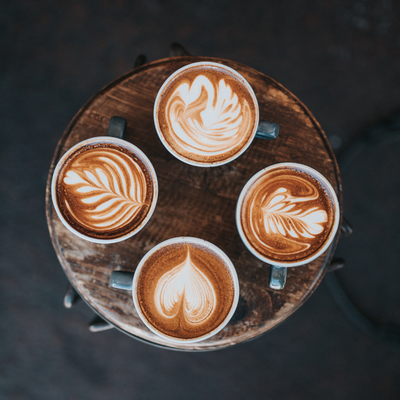This is a close-up, indoor color photograph taken from above, capturing four ceramic mugs of coffee placed in a perfect square arrangement on a rustic wooden table. Each mug contains a latte with unique, intricate designs made from white cream atop the espresso-brown surface. The designs include a spade in the lower cup, a leaf pattern in the left cup, a more circular leaf ending in a heart in the right cup, and a feathery, less distinct pattern in the top cup. The wooden table appears heavily worn, adding to the rustic charm, while the background is a dark, nondescript floor that could be either concrete or tiled, enhancing the focus on the beautifully crafted lattes. The mugs also hint at having light green handles, which subtly stands out against the rich, inviting colors of the coffee and cream.